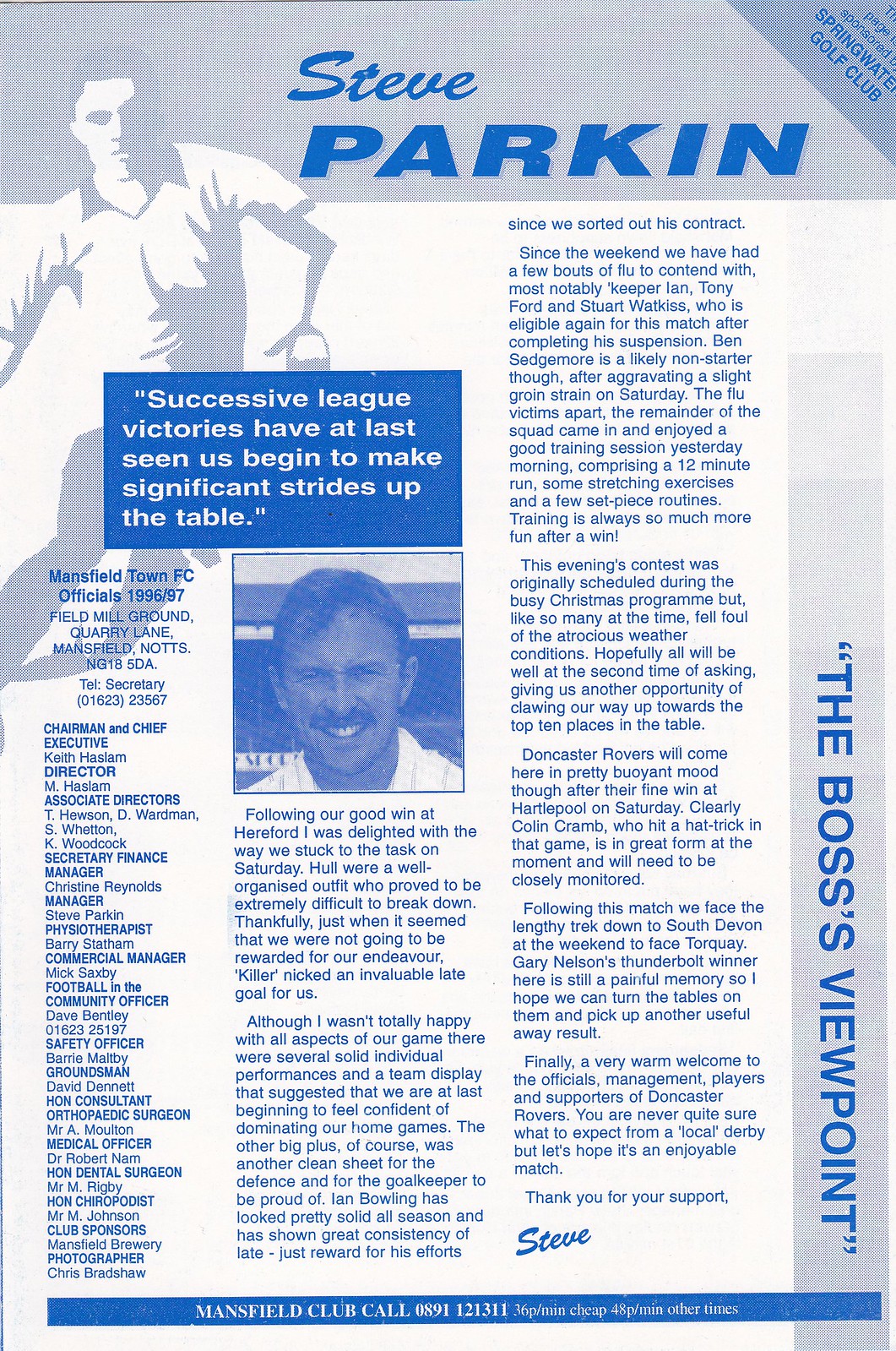This image depicts an informational page from an English football magazine, focusing on Steve Parkin. Dominating the top of the page in bold blue text is his name, "Steve Parkin." The layout includes a shadowy background graphic of a person, presumably Parkin, along with a gray header and a blue footer. A significant portion of the page is dedicated to detailed text arranged in seven paragraphs forming two columns. 

Starting with a notable quote in a blue box, it reads, "Successive league victories have at last seen us begin to make significant strides up the table." Below this, there is a black-and-white photograph of Steve Parkin, identifiable by his mustache. Further blue text follows, summarizing recent games: "Following our good win at Hereford, I was delighted with the way we stuck to the task. On Saturday, Hall wore a well-organized outfit who proved to be extremely difficult to break down. Thankfully, just when it seemed that we were not going to be rewarded for our endeavor, a 'killer' nicked an invaluable late goal for us." The accompanying commentary highlights individual and team performances, suggesting growing confidence in their home games despite some areas of concern.

On the left side of the columns, there appears to be a list of people involved with the football club from the corporate side. On the very right side, a blue vertical band reads "The Boss's Viewpoint." The write-up ends with a note of gratitude: "Thank you for your support," signed by Steve Parkin. At the very bottom of the page, there's a mention of "Mansfield Club call 089 112 1311 at 36 pence per minute, 48 pence per minute at other times," providing contact information presumably for fans or club members.